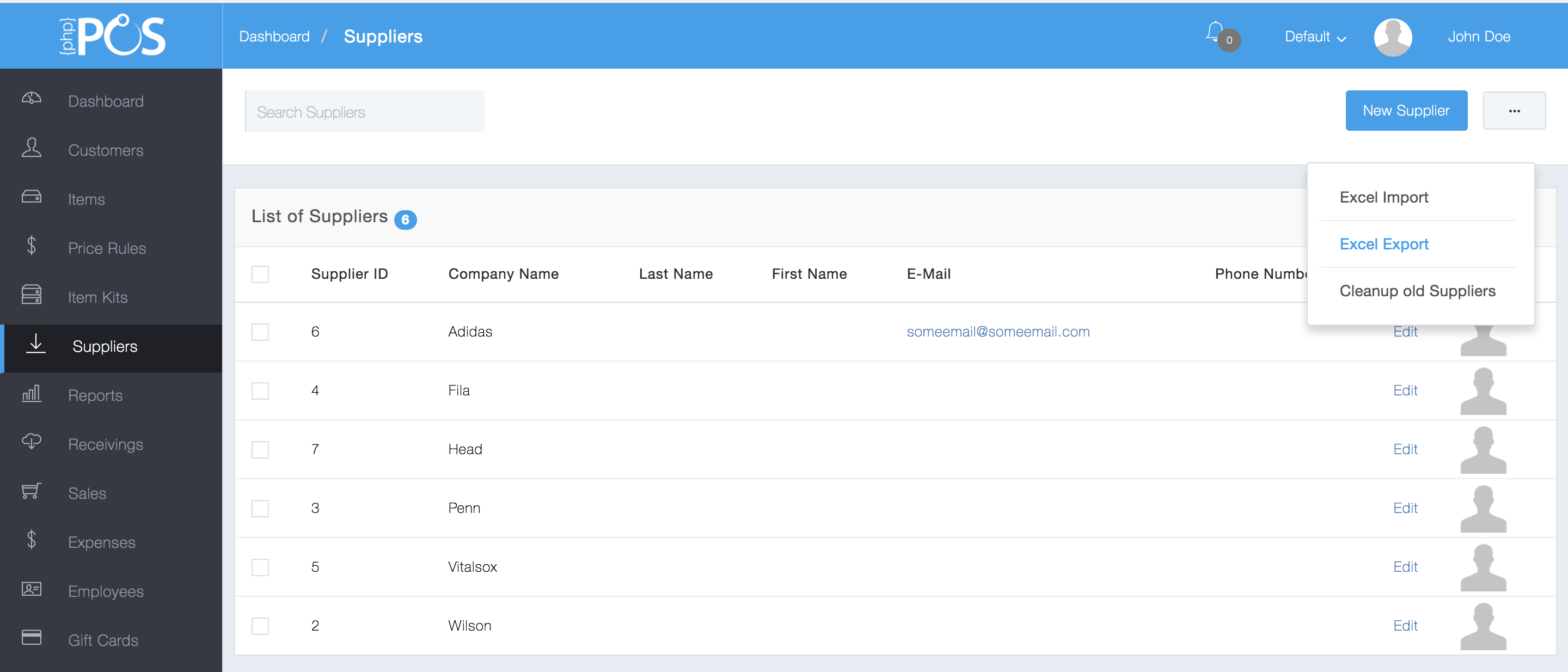In the screenshot from a platform called PCS, the interface is displayed on the 'Suppliers' tab. The header of the page reads "List of Suppliers." Below this, there are columns labeled with numerical ID, company name, contact's last name, first name, and email address. However, the readability is poor due to the use of light gray text on a dark gray background. The sidebar on the left features various navigation options including 'Dashboard,' other indiscernible labels, 'Price Plans,' and the highlighted 'Suppliers' tab. Notably, only the first supplier listed has an email address provided, leaving the email columns for the other entries empty. The design choices make extracting detailed information difficult.